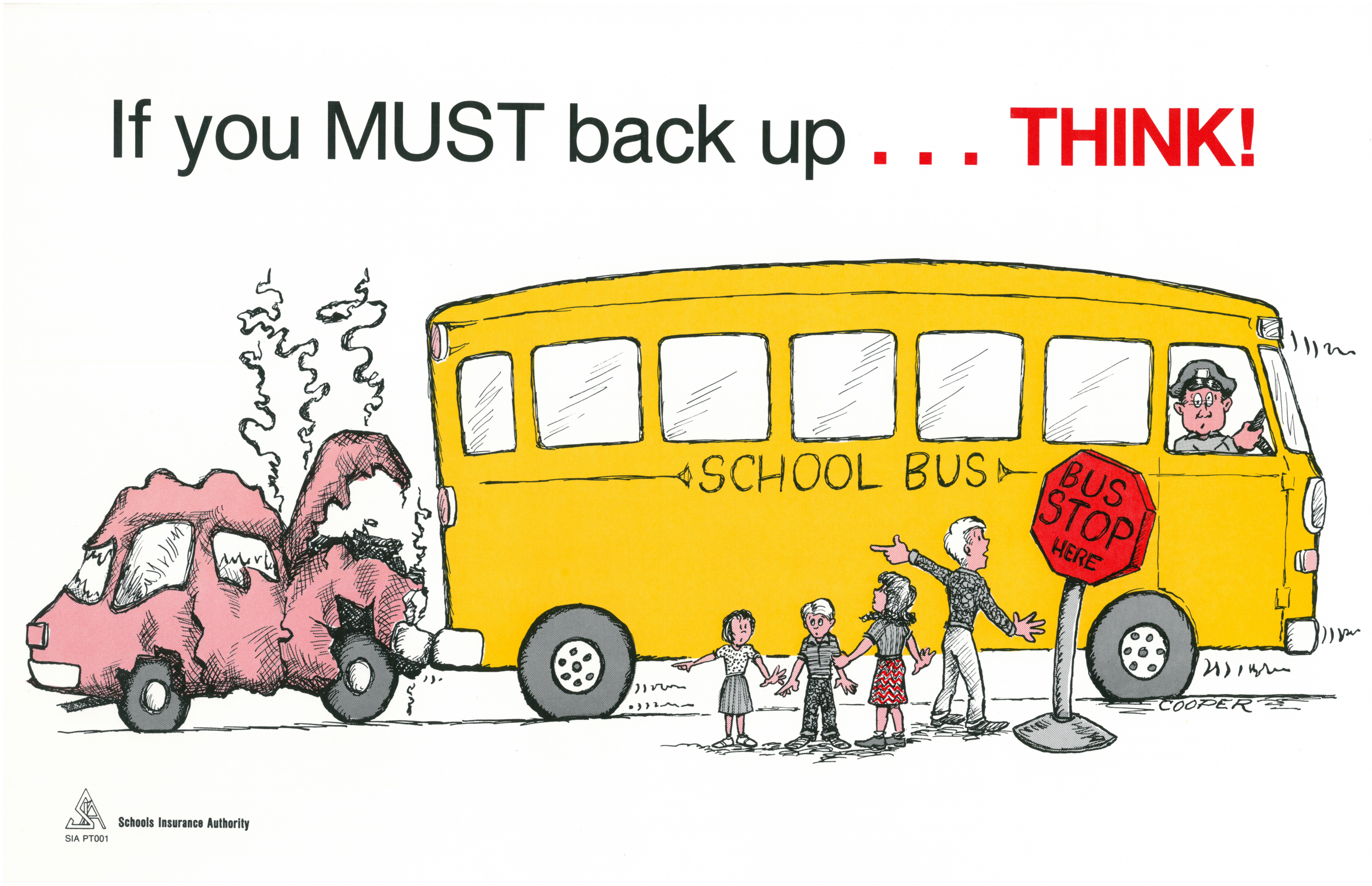In this drawn image, a bold, typed message at the top reads, "IF YOU MUST BACK UP... THINK!" The word "MUST" is in capital letters, while the ellipsis and the word "THINK!" are in a striking red font, emphasizing caution. Below this, a yellow school bus takes center stage, with a confused-looking driver visible inside. The bus has evidently backed into a small red car, likely a Volkswagen, causing significant damage: the front end is mangled, steam is rising from the crumpled hood and radiator, and the windshield and rear of the car are smashed, leaving only the rear bumper intact.

Nearby, at a bus stop marked by a red "Bus Stop Here" sign on a silver pole, stand four people: one adult male and three children (two girls and one boy). The adult, possibly the car owner, appears upset and is pointing towards the wrecked vehicle. The scene is signed by "Cooper" in the bottom right corner and is associated with the School's Insurance Authority, lending it the feel of a public service announcement. The cartoonish style of the illustration adds a slight touch of humor to the otherwise serious message about the importance of caution when backing up vehicles.